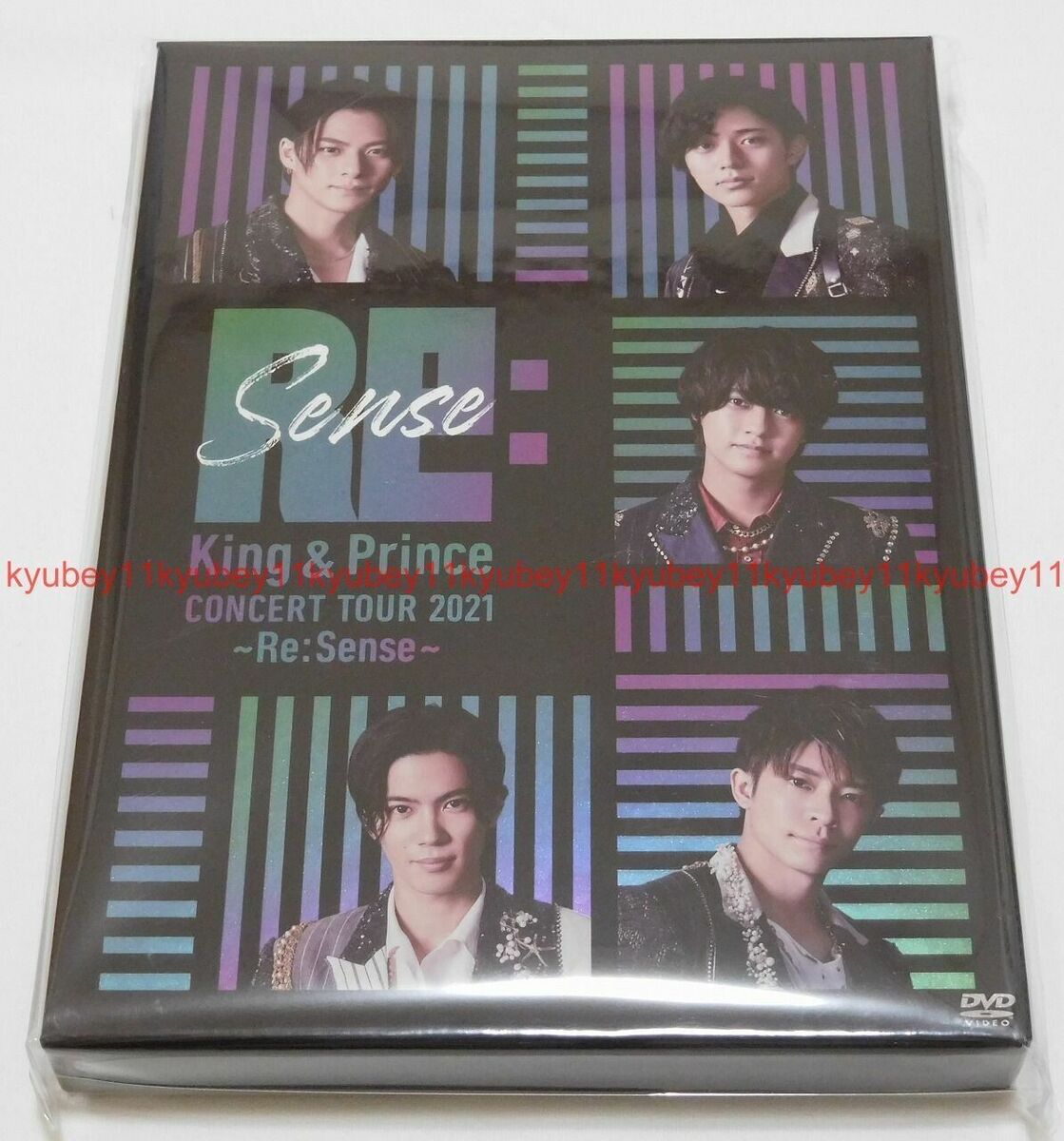The image is a DVD cover with a solid light gray background, lying at an angle on a light gray surface. The cover features a reverse C-shaped arrangement of five small square portraits, each containing a late teen to early 20-year-old attractive Asian young man with dark hair, styled short but falling over their foreheads. They are dressed in dark clothing, adorned with some jewelry, and are set against a backdrop of teal, blue, and purple gradient lines.

The center-left of the cover displays the title "R.E.; sense" with "R.E." in large block teal and purple text, and "sense" overlayed in a smaller white cursive font. Below the title, it reads "King and Prince Concert Tour 2021" followed by another "R.E.; sense." The lower right corner of the cover is marked with a "DVD Video" logo. The entire DVD cover is wrapped in hard, clear plastic.